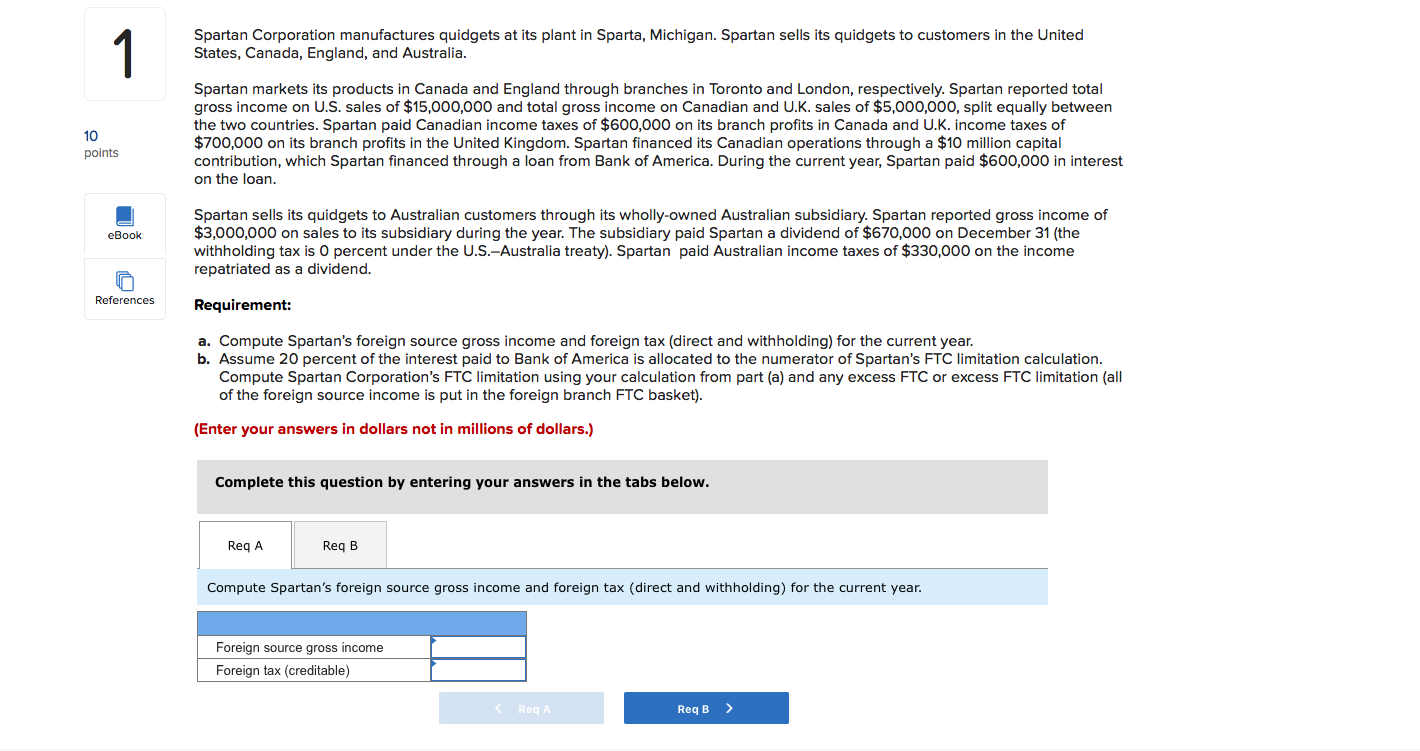Spartan Corporation, an entity involved in the manufacturing and distribution of Spartan products, caters to customers in the United States, Canada, England, and Australia. The corporation markets its products in Canada and England through its branches located in Toronto and London, respectively. Spartan Corporation reported a total gross income of $15 million from U.S. sales and an additional $5 million from sales in Canada and the U.K. 

In terms of tax payments, Spartan paid $600,000 in Canadian income tax and $700,000 in U.K. income tax on its profits derived in these countries. To finance its Canadian operations, Spartan made a $10 million capital contribution, which was financed through a loan from Bank of America. This loan incurred an interest payment of $600,000 during the current year. 

For its Australian market, Spartan sells goods through its wholly-owned Australian subsidiary. During the year, Spartan reported a gross income of $3 million from sales to this subsidiary. Furthermore, the subsidiary paid Spartan a dividend ranging between $670,000 and $730,000, while Spartan paid $330,000 in Australian income tax.

To compute Spartan's foreign source gross income and the associated foreign tax withholdings for the current year, it is necessary to consider the allocation of 20% of the interest paid to Bank of America to the numerator of Spartan’s Foreign Tax Credit (FTC) limitation. The task also involves calculating the FTC limitation using the formula specified in Part 3 and determining any excess FTC or excess FTC limitation, with all foreign source income classified into the appropriate FTC basket. All answers must be presented in dollars, not in millions of dollars, following the requirement to compute the creditability of the foreign tax for Spartan's foreign source gross income.